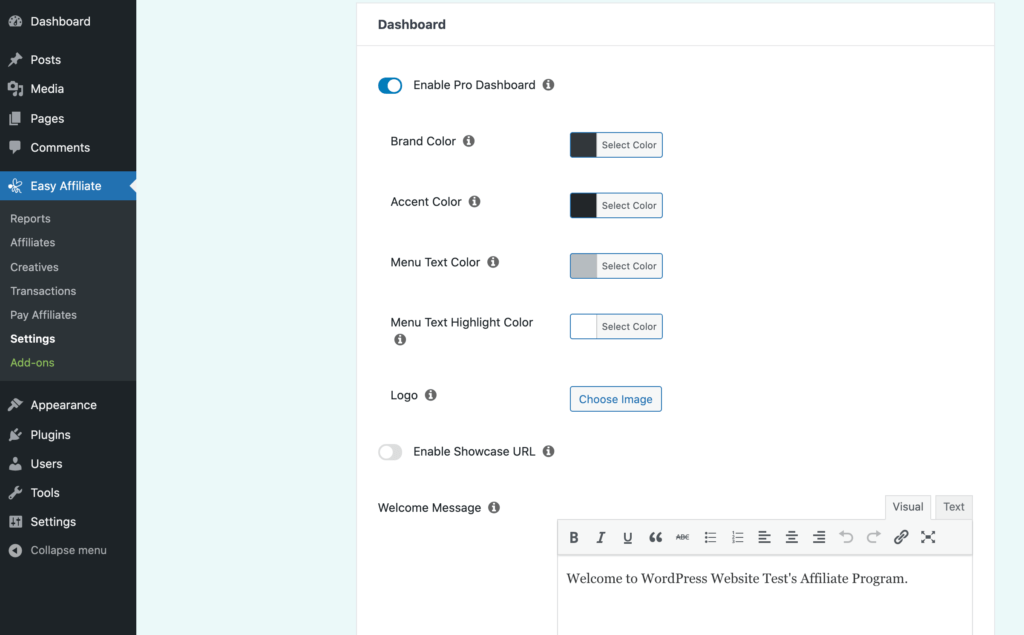**Detailed Description of the Settings Page Interface**

The image illustrates a comprehensive settings page. On the left section, within a dark blue sidebar, there is a vertical menu. The first item in this menu is labeled "Dashboard," displayed in white text, accompanied by an icon of a pedometer. A bit further down, there is an icon of a pin next to the label "Post." Below this, there appears an icon of a camera and a music note symbolizing "Media." Subsequent items include an icon of two stacked squares labeled "Pages," a squared comment bubble icon labeled "Comments," and a bee-like icon with heart-shaped wings that is currently selected. This selected bee icon is highlighted with a cyan blue box, featuring white text inside and a white bee icon with a white arrow pointing to the right, indicating its active status.

Cascading beneath this selected item are additional options: "Reports," "Affiliates," "Creations," "Transactions," and "Pay Affiliates." The option "Settings" is displayed in bold white text, followed by "Add-ons," which is highlighted in green. This section transitions from a light bluish-gray back to dark blue, where further options are illustrated: a paintbrush icon labeled "Appearance," the end of an electrical plug labeled "Plugins," an image of a person labeled "Users," a wrench labeled "Tools," and a dark gray square with two black sliders labeled "Settings."

At the bottom, there’s a gray circle with a dark blue arrow pointing left, labeled "Collapse Menu."

To the right, occupying the main portion of the page, is a cyan blue background containing a large white rectangle. The top of this section features a dotted gray border with the label "Dashboard" in bold black text. Directly below is a slider switched to the right, indicating it is active. The background on the left of this slider is dark blue. The phrase "Enable Pro Dashboard" in black text accompanies a gray circle with a white "i" in its center, providing information. Following this is the "Brand Color" option with a drop-down menu currently showing dark blue or black. 

Next, "Accent Color" is listed with the same informational circle, which appears to be more black, thus confirming the first selection was dark blue. "Menu Text Color" is set to dark gray, and "Menu Text Highlight Color" is set to white. Below that, the section labeled "Logo" provides an option to "Choose Image."

Following this, there is another slider set to "Off," indicated by a white circle on the left and a dark gray background on the right. This controls the "Enable Showcase URL" function. At the bottom, the "Welcome Message" section is shown with a smaller rectangle bordered in dark gray, featuring various text-editing tools: bold, italics, underline symbols, quotation marks, ABC numbering, bullet points, text justification options (left, right, or center), refresh, undo and redo icons, hyperlink insertion, and an "X" symbol for expanding or modifying the view. The current message reads, "Welcome to WordPress website test affiliate program."

This detailed caption provides clarity and structure to the described settings page layout.